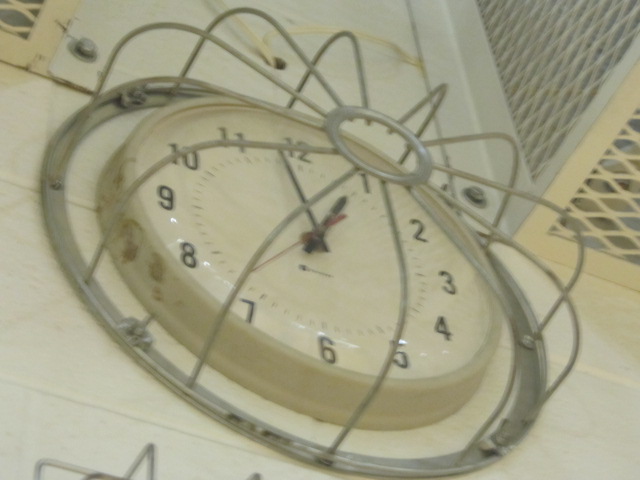This image features a clock mounted on a white cinder block wall. The clock is encased in a protective silver metal cage, which is securely bolted to the wall. The cage has curved, thin metal bars that extend over the front of the clock, presumably to prevent it from being damaged or knocked off the wall. Similar protective cages are often found in environments like gymnasiums in schools. The clock itself is off-white with a white face. It displays the time as 12:58, with black hour and minute hands and a red second hand. The clock face is marked with numbers from 1 to 12 in a clockwise arrangement, and there are four small hash marks between each number for precise timekeeping.